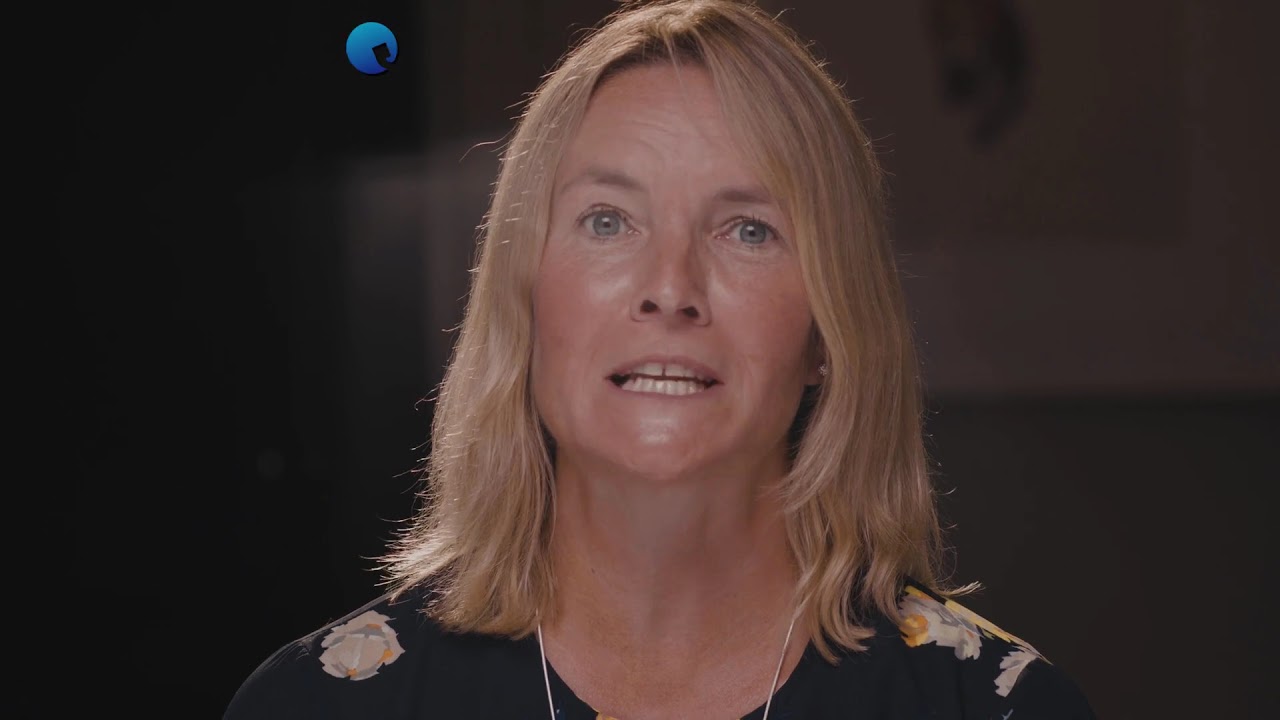The image shows a Caucasian woman with shoulder-length, straight blonde hair parted slightly to the left of center. She has pale blue eyes, with the eye on the left side of the image open just a bit more than the one on the right. The woman has a slight gap between her two front teeth, and her mouth is partially open, revealing her top and bottom teeth, with the bottom teeth angled slightly inward. Her face and neck have a rosy hue, with some reflections on her forehead and under her eyes indicating glossy skin. She is wearing a dark-colored top adorned with floral designs on the shoulders. Around her neck, there is a necklace, though the photo cuts off just below the neckline, obscuring detailed view of the necklace. In the background, particularly on the upper left, there is a blue circle that has lighter shading at the top and darker shading at the bottom, interrupted in the center by a square shape. The left part of the background is dark and becomes increasingly pitch black, while the right is slightly more illuminated, revealing vague, indistinct objects.